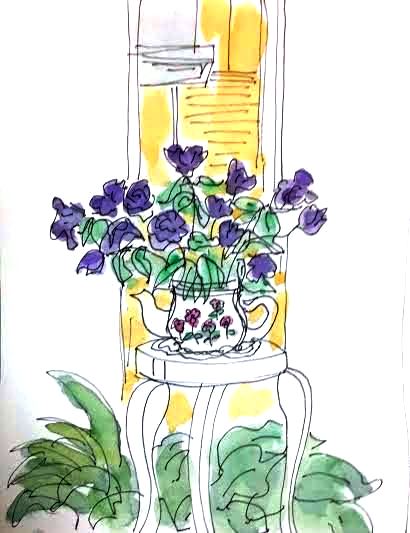This artwork features a meticulously detailed black ink hand drawing of a teapot, evocative of a traditional jug, adorned with intricate floral designs. Emerging from the teapot are elegant, purple-stemmed flowers with lush green leaves. The teapot is gracefully perched atop an unpainted flower pot stand. Accentuating the base of the stand are additional green leaves, adding a touch of vibrancy to the composition. The line drawing has been partially colored with watercolor, bringing life to the flowers and foliage. Behind the teapot and stand, a yellow-painted spiral staircase serves as a whimsical backdrop, creating a dynamic and inviting scene. The teapot itself, as well as the stand, remain uncolored, standing in striking contrast to the vividly painted elements surrounding them.